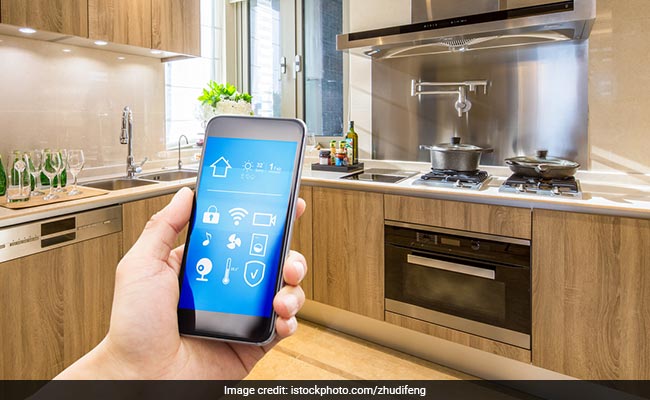The photograph captures the interior of a home kitchen with wooden cabinets both above and below the counter, and a window in the background. The kitchen has an L-shaped layout; on the left side, there is a dishwasher beneath the counter with several glasses placed on a mat above it. Adjacent to the dishwasher, there is a two-part sink. The other side of the L features a built-in stovetop and oven, complete with a pasta pot filler overhead. The stove has some pots on it, and to the right of the sink, there are items that look like olive oil bottles. In the foreground, a person's left hand holds a black smartphone. The smartphone displays a blue screen filled with white icons related to Internet of Things devices, arranged in a 3x3 grid. The icons include a house, temperature, a lock, a Wi-Fi symbol, two camera symbols, a music symbol, a fan symbol, a washing machine symbol, a temperature symbol, and a shield with a checkmark. The phone is positioned slightly off-center to the left, and there is an image credit banner at the bottom of the photo, indicating iStockphoto.com.